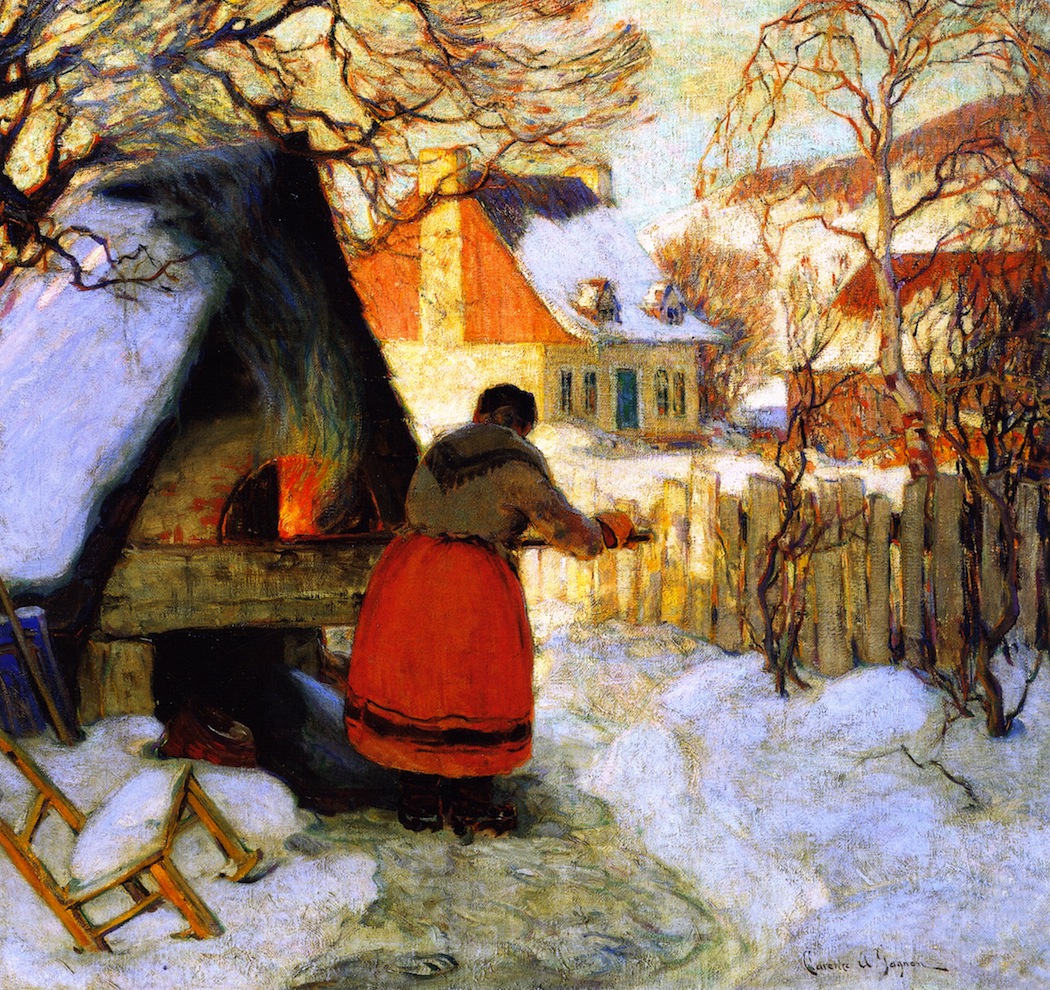In this evocative painting, a woman stands at the center of a wintery farmstead, tending to an outdoor fireplace hearth with a long stick, as if cooking something. She is dressed in a red skirt and a brown blouse with a shawl or scarf draped over her shoulders. Her attire stands in contrast to the white snow that blankets the ground and the objects around her. Beside her, a rocking chair, yellow and dusted with snow, leans to the left. 

The hearth emits vivid red and orange flames, with smoke curling up into the gray-blue, molted sky. Surrounding the scene, there are gnarly, leafless trees and a wooden picket fence. In the background, a beige and brown house with a tin and red roof adds a touch of rustic charm. The painting, reminiscent of Van Gogh's flowing style but less abstract, captures a tranquil yet dynamic winter day on a farmstead, where the presence of fire provides a warmth against the snowy backdrop. The artist's signature is discreetly placed below, indicating the creator's personal touch.